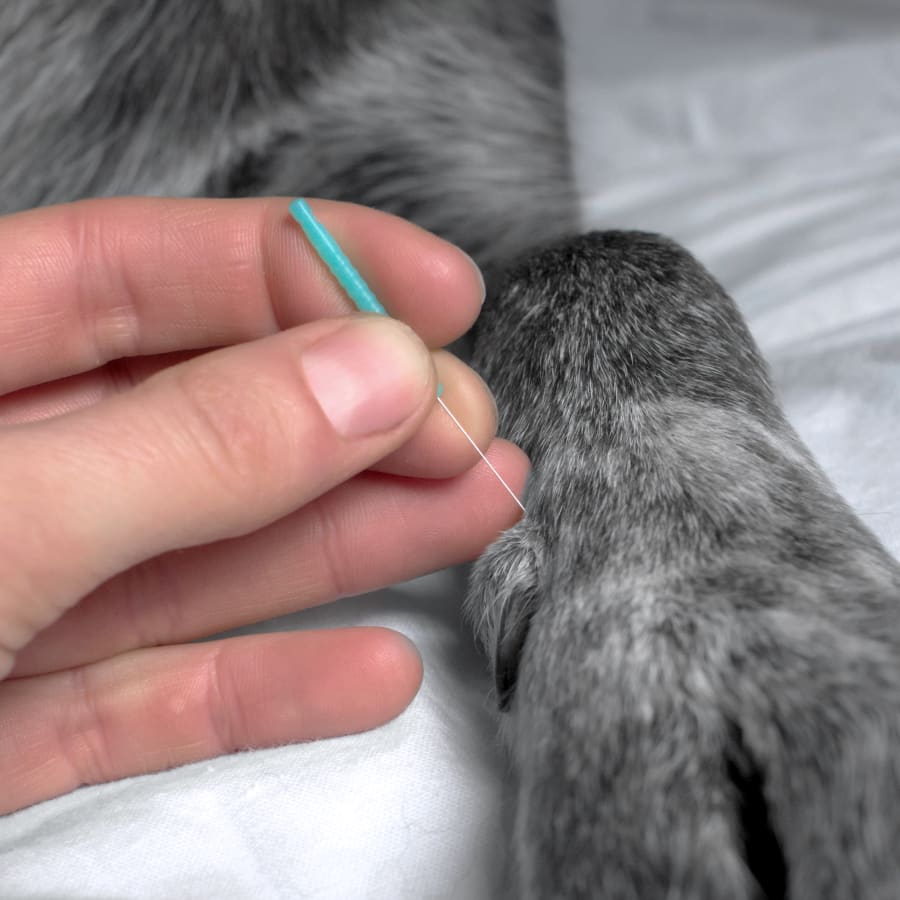This close-up image depicts a veterinary procedure involving a dog with gray and white fur. The photograph centers on a fair-skinned human hand holding an acupuncture needle with a turquoise-blue handle and a thin, silver needle. The needle is being gently inserted into the dog’s paw, specifically near a dark, black nail, which adds context to its positioning in the image. The dog’s leg stretches diagonally from the bottom right towards the top left, resting on a textured white blanket that covers part of the dog's body. The animal's fur, a mix of very dark gray and lighter almost white patches, suggests it is a breed with short hair. The scene is likely set in a veterinary office given the clinical nature of the setup and the white blanket underneath the dog for support. The focus remains on the interaction between the human hand and the dog’s paw.